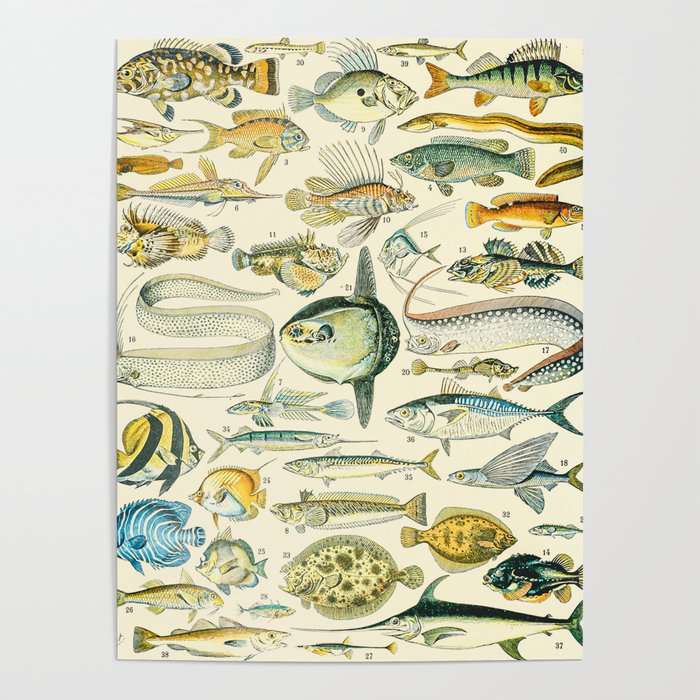This highly detailed infographic showcases a variety of fish species through realistic drawings. Numbered from 1 to 32, the fish are depicted without any additional text, emphasizing their visual differences and similarities. The illustrations feature an array of fish, including eels, a swordfish or marlin, a flounder, and an angelfish, as well as a tuna and a flying fish. The vibrant colors range from yellow with vertical black stripes to blue and white swirls, and patterns from swirls to solid colors. Despite their differences, all the fish share common features like fins and tail placements. Set against a clean white background, some fish swim left, some right, and they vary greatly in size and shape, making this an informative diagram for identifying different types of fish.